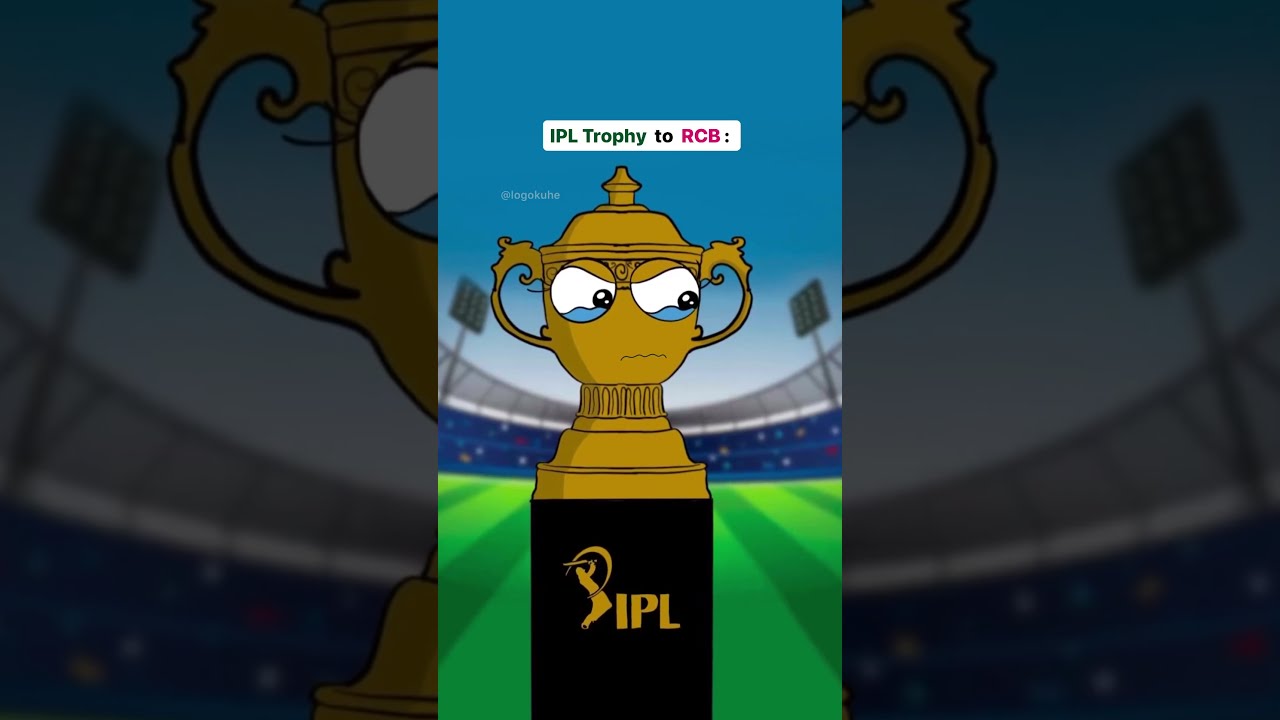The image consists of a horizontally rectangular digital collage depicting a sporting scene. The main focus is a vertically rectangular central panel featuring a gold trophy with two handles, set on a black base. The trophy has anthropomorphic features, with large, expressive eyes looking to the left, and blue tears welling up in the bottom of the eyes. Above the trophy, in capital letters, it says "IPL Trophy to RCB," with "IPL" in gold and "Trophy to RCB" in pink text.

The background illustrates a faded, blurry arena with a blue sky and different colored dots representing people in the stands. There are two gray light posts, one on each side of the field, which is vivid green. The trophy appears to have a slightly cartoonish or caricatured style, adding a whimsical feel to the image.

Around this central image, there are two vertically rectangular panels on the left and right, each showcasing the same arena scene but as a separate and more zoomed-out backdrop that forms a continuous image when viewed as a whole. The left and right panels are identical to the central scene but extended outward, giving a panoramic feel to the overall composition.